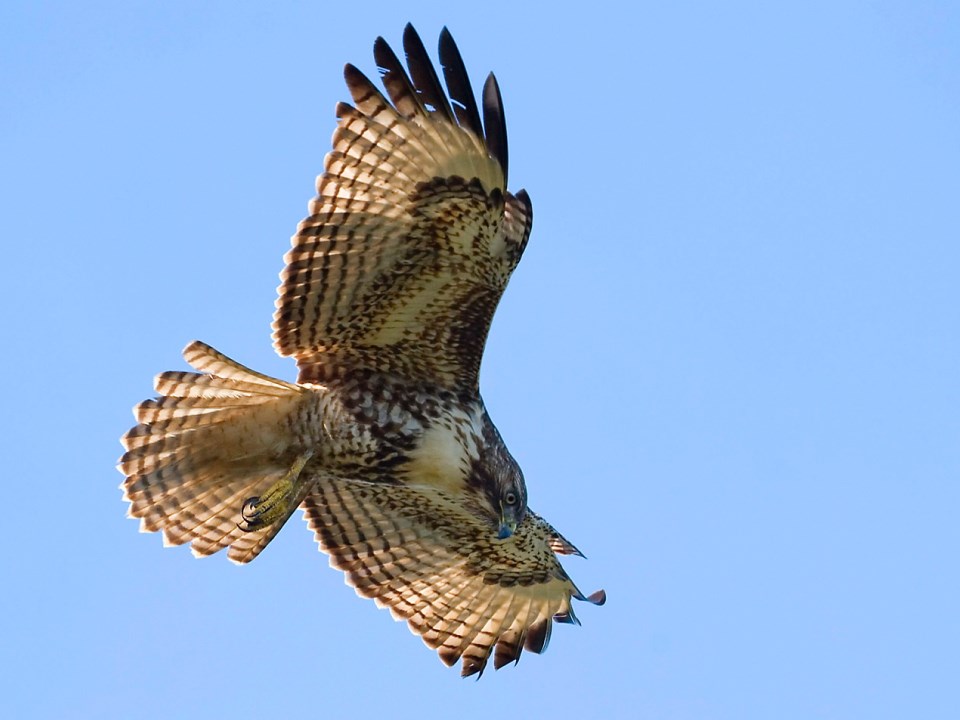The image captures a majestic hawk soaring through a cloudless, light blue sky. The bird has its wings fully outstretched, showcasing a striking pattern of black and white speckles, with dark brown tips on the wing feathers. The underside of its wings is predominantly white with distinctive brown stripes and spots peppering the inner parts. The hawk's body is a blend of creamy white and brown, accented by a pure white area just below its neck. Its tail feathers are fanned out, displaying a similar brown-striped pattern on a white background.

This hawk, with its bright yellow legs and feet curled under its body, appears to be in a hunting mode, as its head is angled downward with intense yellow eyes indicating focus. The beak is a dull yellow with a dark tip, curved into a formidable shape perfect for hunting. Notably, the bird clutches a cylindrical object in its long, black-tipped talons, adding an element of intrigue to the scene. The overall image presents an exquisite, dynamic snapshot of the hawk's elegant yet powerful presence in flight.